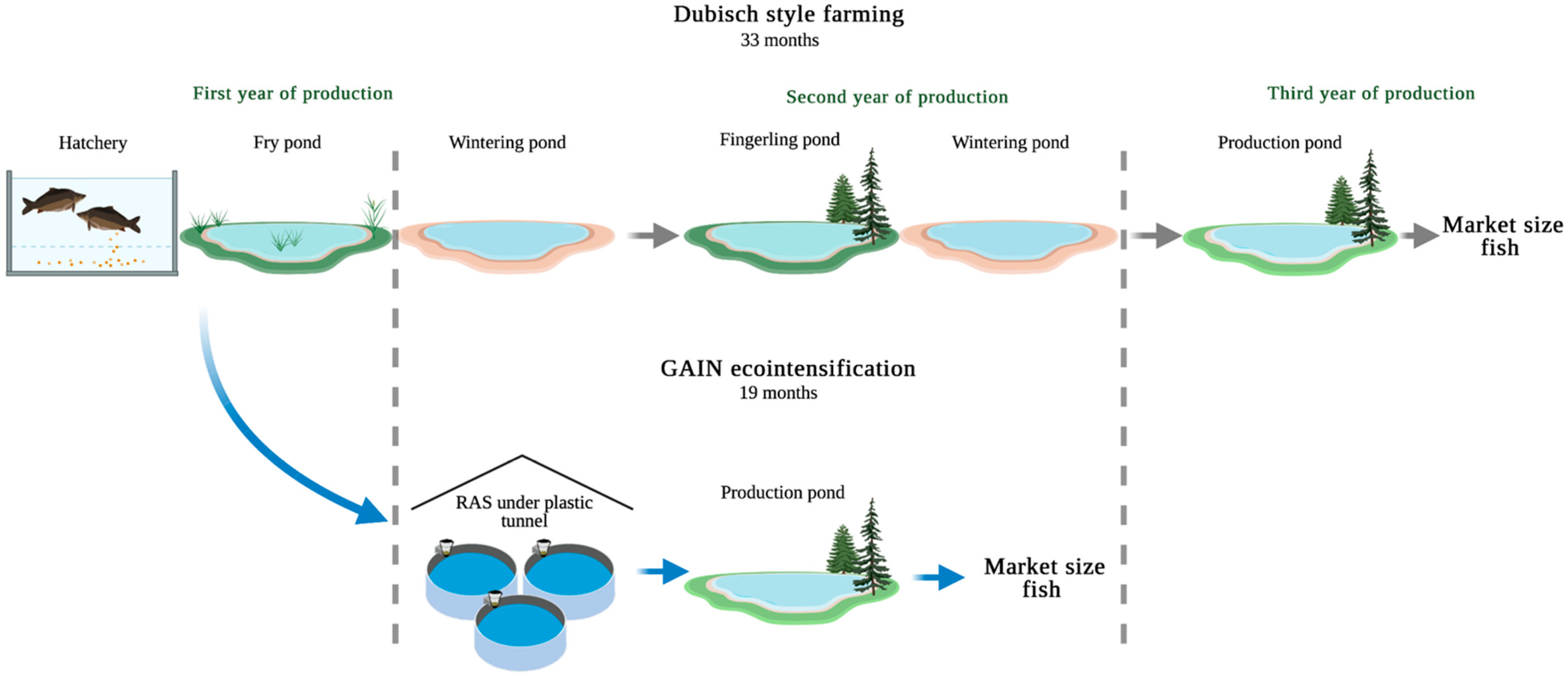This detailed diagram illustrates the Dubish Style Farming method with a timeline of 33 months. The top of the image prominently features the title "Dubish Style Farming" in black serif-style font. The diagram is structured into different stages of fish farming, beginning on the upper left with the hatchery, labeled "First Year of Production," and progressing through to the right with various ponds. 

In the first year, the diagram showcases a hatchery with two fish illustrated in a tank, followed by a "Fry Pond" depicted with light turquoise water, and a "Wintering Pond." The second year moves on to a "Fingerling Pond" amidst dark green trees, another "Wintering Pond," and into the third year with a "Production Pond." The culmination of this cycle is indicated by the term "Market Size Fish."

The bottom section of the diagram emphasizes "Gain Eco-Intensification" over 19 months, featuring "RAS under Plastic Tunnel," with three circular tanks filled with water. Arrows guide the viewer through the sequence from the production pond to the market-size fish, highlighting the continuity and organization of the farming process.